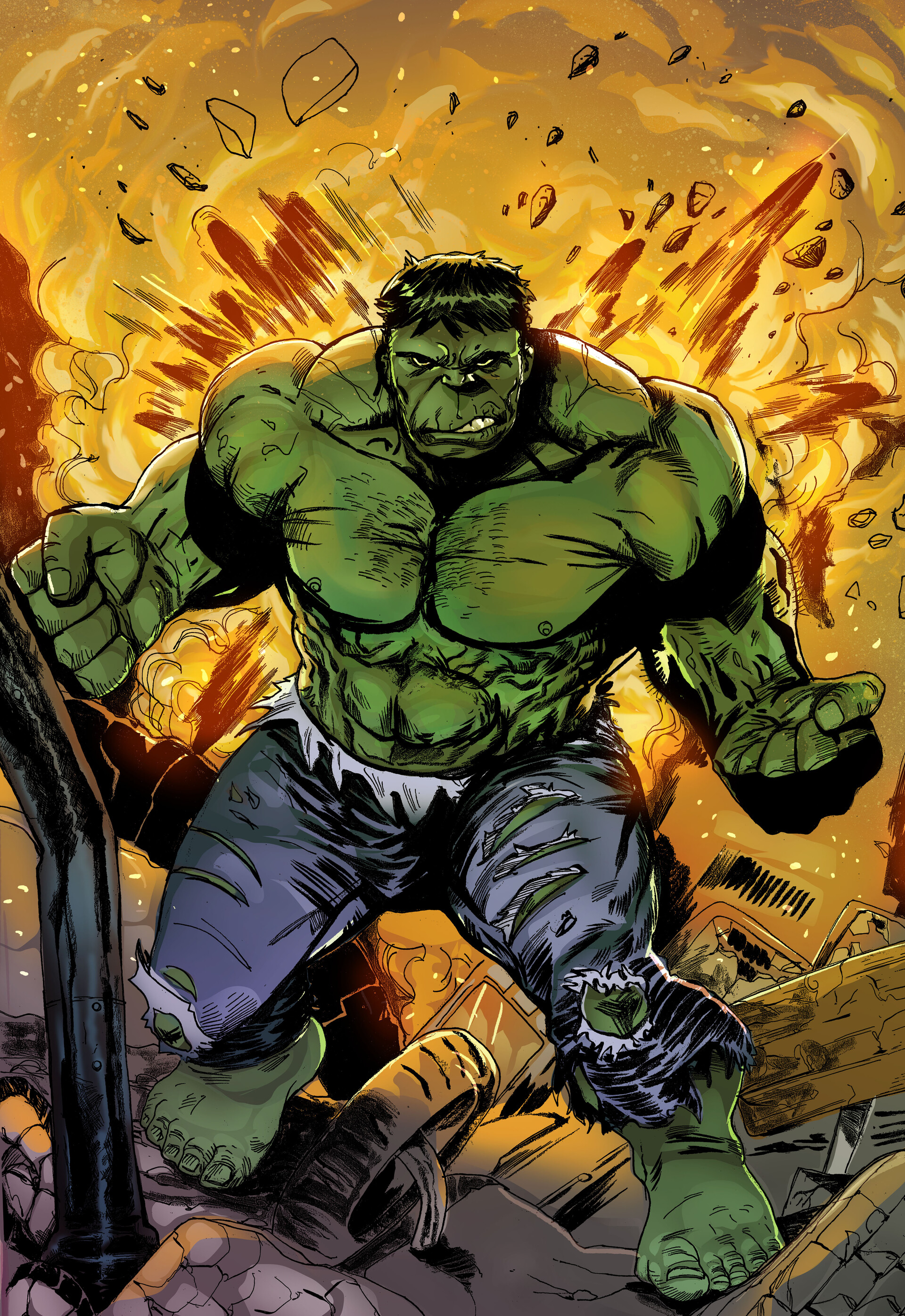The image is a detailed color illustration of the Incredible Hulk, depicted in portrait mode. The character stands out with his green skin and immense, chiseled muscles, exuding formidable strength. He is wearing tattered purple pants that are ripped at the thighs and knees, accentuating his powerful physique. His clenched fists and imposing stance suggest he is displaying his might, stepping purposefully toward the viewer. The Hulk's black hair frames an angry, snarling face with teeth bared and eyes glaring intensely, adding to the character's intimidating presence.

The chaotic background reinforces the theme of destruction, with vibrant, fiery hues of yellow, orange, and red suggesting an explosion. Flames and debris like wood, rock, and scattered electronic parts lie under his massive feet, creating a scene of devastation. The overall atmosphere of the drawing is one of raw, unstoppable power, embodied by the enraged Hulk, standing against a backdrop of carnage and fire.